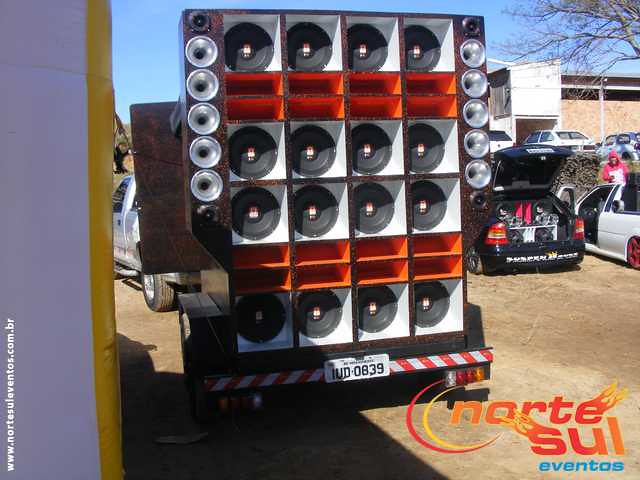This promotional graphic for Norte Sul Eventos prominently features the company's branding with orange, flame-accented text spelling "Norte Sul" and blue letters for "Eventos" in the lower right corner. Their website, www.nortesuleventos.com.br, is written vertically on the left-hand side. The photo depicts the rear view of a trailer mounted with an impressive array of black loudspeakers in white casings, boasting four rows of four large speakers. Below these are additional circular speakers—five on each side. The trailer is connected to a silver pickup truck and sits in a parking lot that also contains two street race cars, each equipped with sizable speakers in their hatchbacks. The background features a building, parked cars, a person in a red hoodie with white lettering, an elevated shed that might serve as an announcer's booth, and trees under a blue sky. The white license plate on the trailer reads IUD 0839.